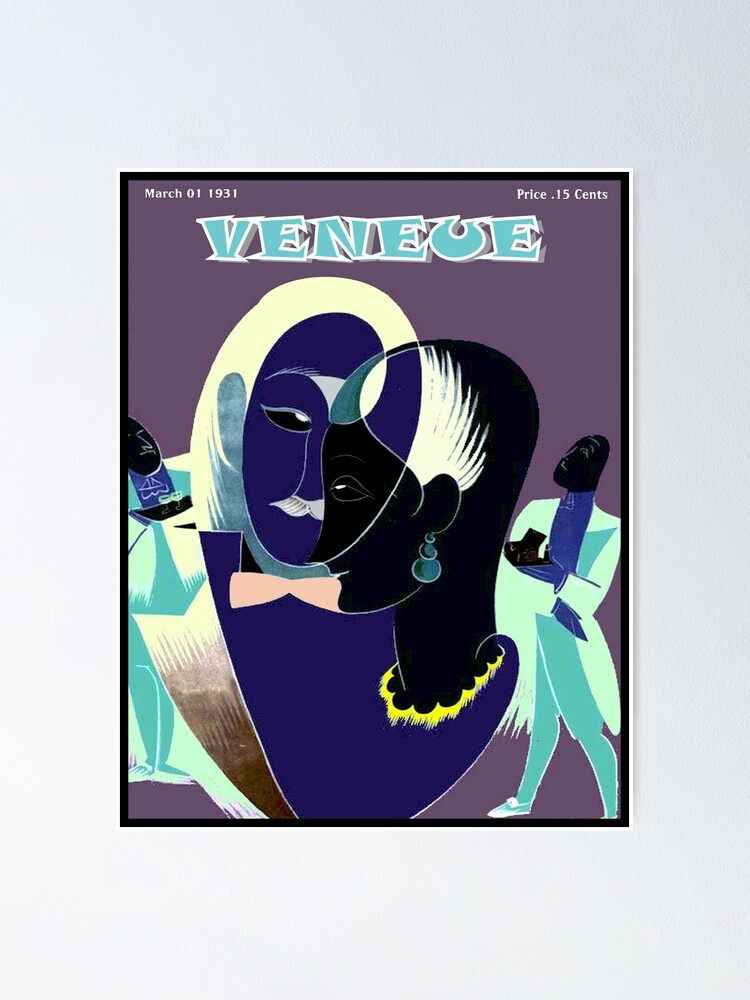The image features a portrait-oriented magazine cover titled "Venue," spelled V-E-N-E-U-E, in three-dimensional turquoise-green lettering with a white outline. It is set against a grey background that transitions from a slightly lighter grey at the bottom left to a subtle silver hue at the top right. The grey is applied more thickly at the top and bottom edges than the sides. The cover is dated March 1, 1931, in the top left corner, with the price indicated as 15 cents in white text on the top right. Framing the cover is a thin black border.

At the center of the magazine cover, there is an intricate, modernistic artistic interpretation featuring abstract, geometrically-styled figures. Dominating the middle of the cover are two intertwined heads, almost forming the shape of a heart. 

On the right, the female figure has a black face looking left, adorned with what appears to be a white feather above her ear, turquoise-green earrings, and a yellow, fluffy collar at the base of her neck. Her features are accented in a highly stylized form.

To the left, the male figure has a blue face with a white mustache, yellowish hair, green skin on the ears and chin, and a blue chest with a beige bow tie. 

On either side of these central figures are humanoid shapes featuring distinctive attire: A server or attendant in a white suit with light blue pants on the right, holding an ambiguous black object resembling an upside-down mushroom. Completing the composition is a rich, wine-purple background.